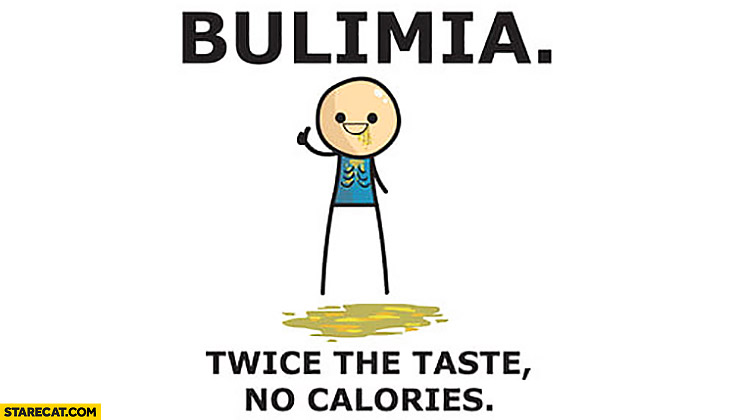This is a detailed cartoon illustration with a distinctive shock value. The central figure, a smiling stick figure with black eyes, is depicted mid-vomit, giving a thumbs-up with one hand. The character, of Caucasian complexion, is wearing a blue shirt that's stained with a mixture of green, yellow, and orange vomit, which is also pooled on the floor in front of it. The character's spindly black legs contrast strikingly with its body, appearing longer than its torso. Above the figure, bold black capital letters spell out "BULIMIA," and below, the tagline reads "TWICE THE TASTE, NO CALORIES." The entire scene is set against a stark white background, with a yellow banner in the bottom left corner showcasing the website name "staircat.com" in black text.